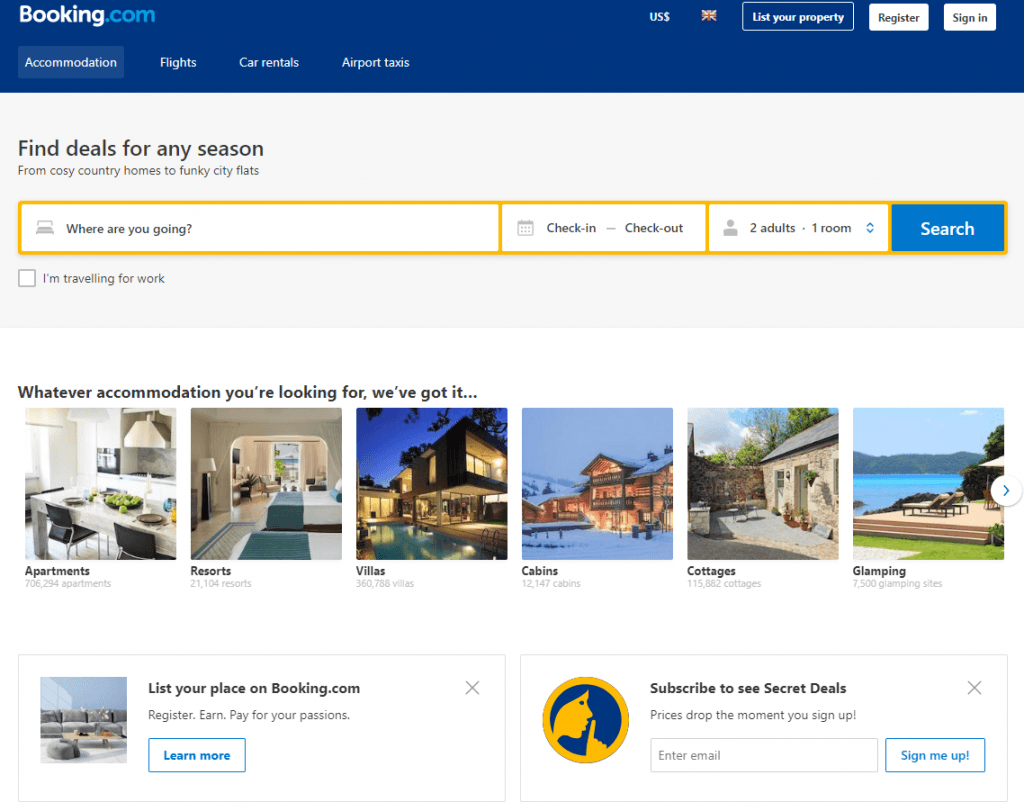This image captures a detailed view of the Booking.com website's homepage. At the top, there is a dark blue border featuring the Booking.com logo on the upper left, with 'Booking' written in white and '.com' in blue. To the right of the logo, there are three buttons: "List your property," "Register" (in white), and "Sign in" (in white).

Below the header, there are several tabs: "Accommodations," "Flights," "Car Rentals," and "Airport Taxis." A prominent gray rectangle is positioned right underneath these tabs, featuring the text "Find deals for any season." Within the gray rectangle, there are three yellow boxes. The first box asks, "Where are you going?" The second box is designated for "Check-in" and "Check-out" dates. The third box pertains to the number of people and rooms needed. Adjacent to these yellow boxes is a blue "Search" button.

Beneath this search section is a white background area with a heading that states, "Whatever accommodation you're looking for, we've got it." Below this heading, there are six square image boxes displaying different types of accommodations: Apartments, Resorts, Villas, Cabins, Cottages, and Glamping. Each image corresponds to its label, showcasing a scene representative of its type.

At the bottom left of the page is a section prompting users to "List your place on Booking.com" with an accompanying "Learn more" button. To the right of this section, there is an invitation to "Subscribe to see secret deals," along with a box for entering an email address and a "Sign me up" button.